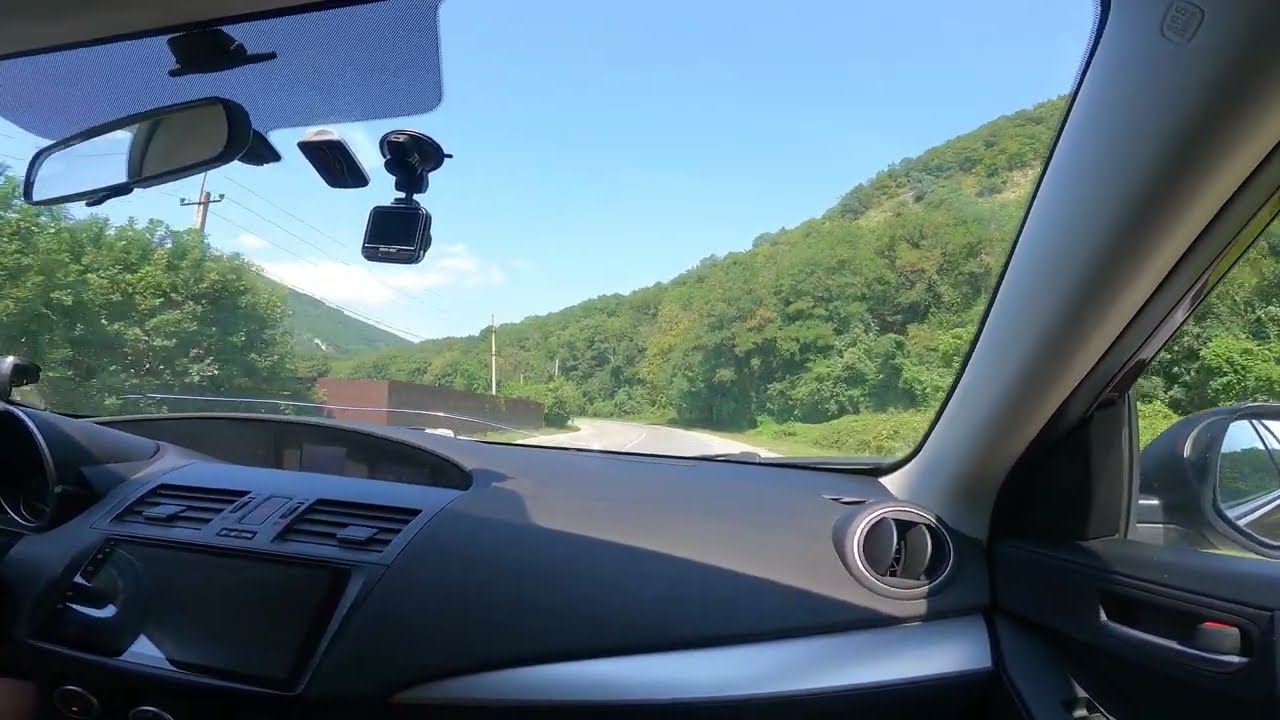The photo captures the view from the passenger side of a car. Inside the vehicle, the dark gray and silver dashboard is prominently featured, with an electronic display at the center of the console and multiple closed air conditioning vents above it. A small recordable camera is mounted on the windshield. Looking through the windshield, the road ahead is light gray with a solid white line in the center denoting the lanes. To the left of the road, a tall brown fence runs along with several wood telephone poles supporting black wires. Behind the fence, a low, potentially one-story brown building can be partially seen before the road curves away. To the right of the road, a steep slope is covered with dense green vegetation and trees. The weather appears to be clear, with a light blue sky complemented by light white cloud coverage. In the distance, more hills and thick green foliage rise up, giving a sense of depth to the landscape.